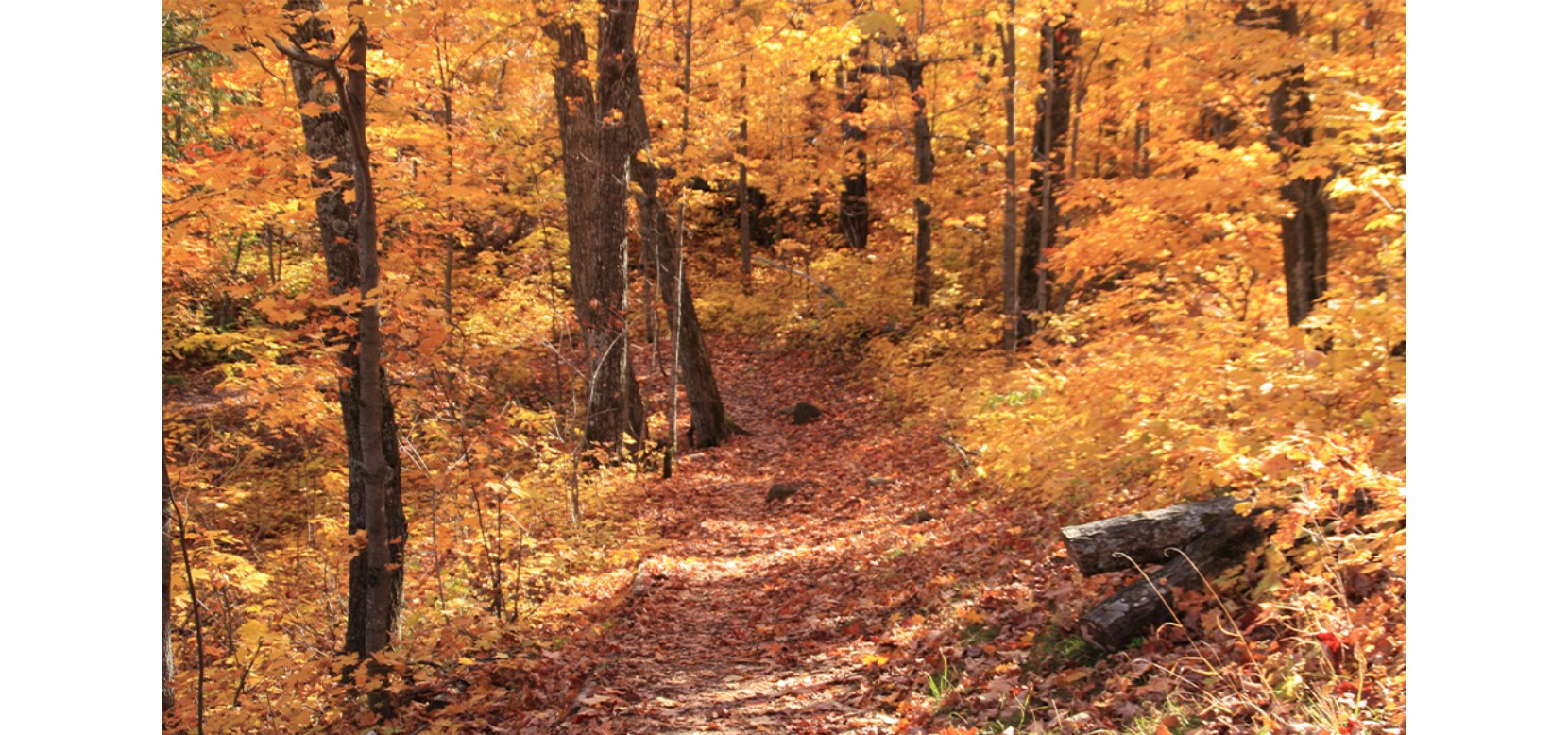This photograph captures a serene forest scene, dominated by the vibrant colors of autumn. In the center of the image, there is a narrow, brown dirt path lightly strewn with dry and decaying leaves, leading invitingly through the woods. On either side of the path, dense clusters of trees with dark brown trunks rise, their foliage a stunning array of yellow and orange hues, creating a canopy that filters the sunlight. The abundant leaves not only blanket the trail but also obscure much of the forest floor, contributing to a sense of depth and enclosure. The sunlight pierces through the foliage intermittently, casting dappled patches of light along the path, accentuating the beauty of this tranquil autumn landscape, ideal for hiking or exploring.